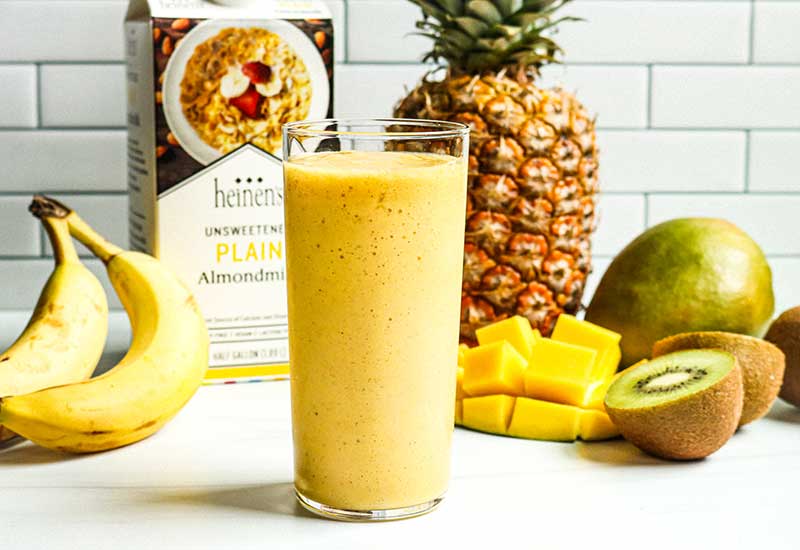In the foreground of this kitchen scene, a tall glass filled nearly to the brim with a golden yellow smoothie takes center stage. Set against a backdrop of white subway tiles with darker grout, the display features an array of carefully arranged ingredients. Behind the glass, a halved kiwi reveals its vibrant green interior next to small, neatly diced cubes of pineapple. A whole pineapple and a full kiwi stand tall, accompanied by a carton of unsweetened plain almond milk. Two bananas, still attached and leaning slightly to one side, rest beside these elements. Additionally, a whole mango and a partially cut mango add to the colorful assembly. This well-curated setup showcases the fresh components that have been blended into the smoothie, providing a visual recipe of the delicious beverage in the glass.